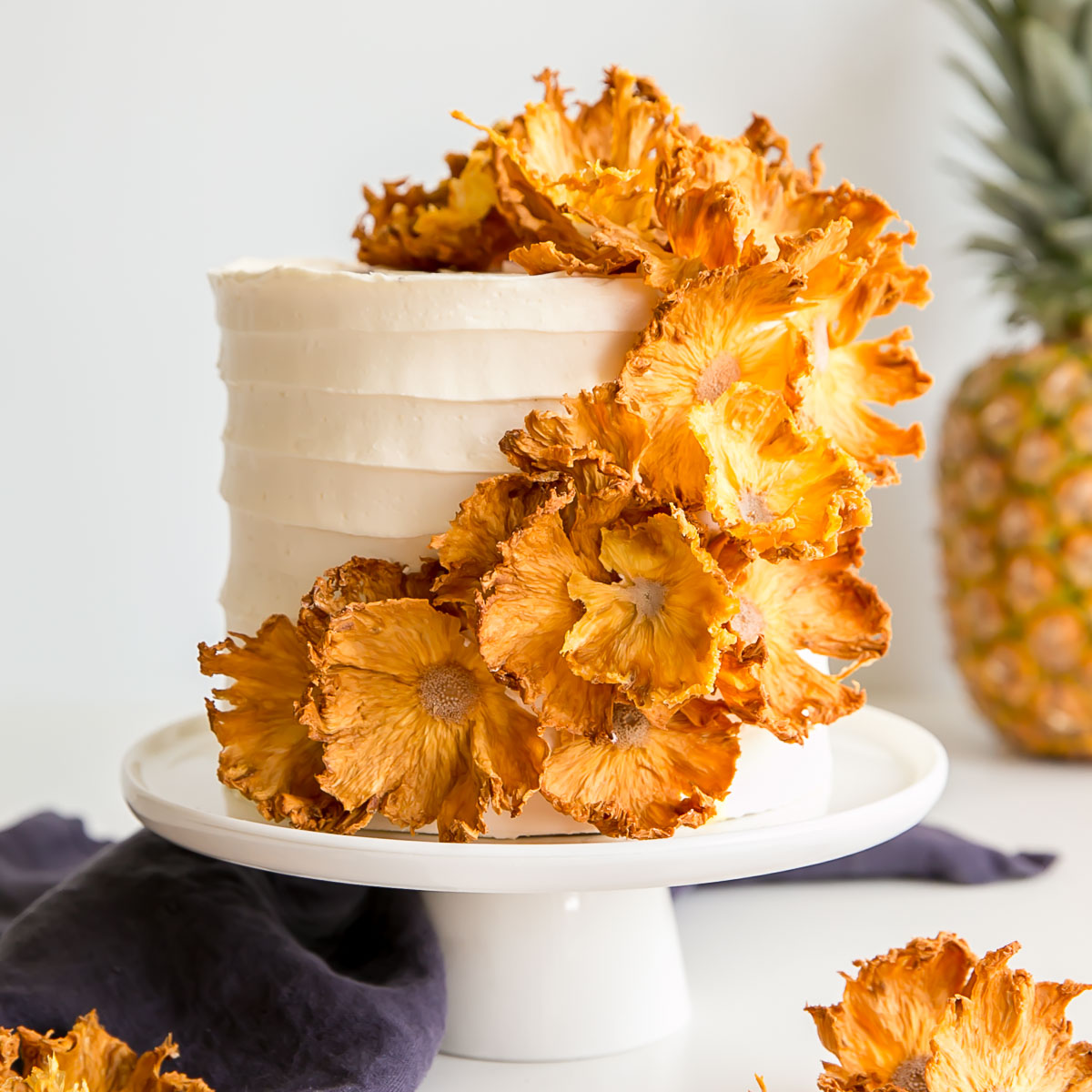The photograph features a tall cake with white, swirled frosting, prominently displayed on a white glass or plastic pedestal. The cake is adorned with brownish-gold dried flowers that cascade from the top, down the right side, and around towards the bottom left. This arrangement creates an elegant, natural aesthetic. The pedestal sits on a white marble table, where a gray dried flower and a blue-gray cloth—possibly a towel—are also visible. The scene is set against a very pale gray or cream-colored background. On the right-hand side, a pineapple with its yellow body and green top is visible, though it is blurred, making it a subtle part of the background composition. The overall setup exudes a refined and artistic presentation, with the dried flowers and decorative elements enhancing the sophisticated look of the cake.